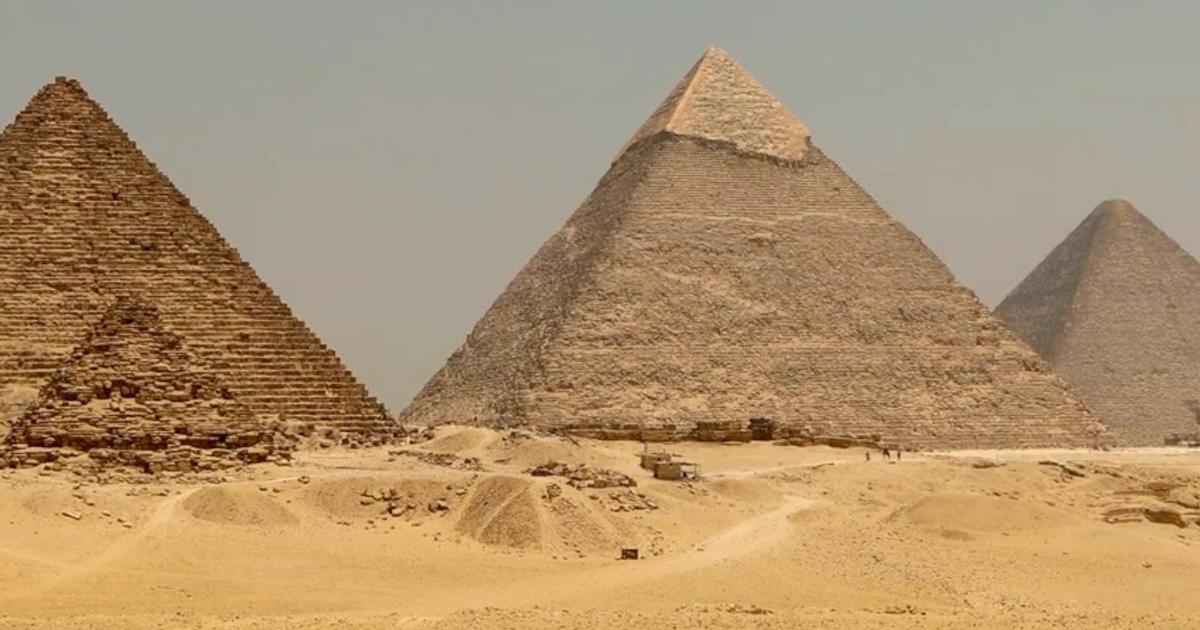This detailed color photograph in landscape orientation showcases the pyramids of Egypt under a gray, gradient sky that darkens towards the top. The central subject is the Great Pyramid, the largest of the three, distinguished by a lighter tan stone at its summit, which forms an irregular shape due to erosion. Its surface is worn, revealing a rough, gray, rocky texture. To its left stands another pyramid, notable for its damaged triangular section at the base, where the stepped layers have crumbled into a heap of scattered rocks. The pyramid on the right, slightly recessed, appears smaller and exhibits a grayer tone. The foreground is covered in yellow desert sand, interspersed with pathways, roads, and tiny human figures that emphasize the monumental scale of the structures. A smaller pyramid-shaped object lies in front of the left pyramid, adding to the scene’s complexity. This realistic photograph captures the historical grandeur of the deteriorating pyramids, framed by the stark desert landscape and illustrating the passage of time.